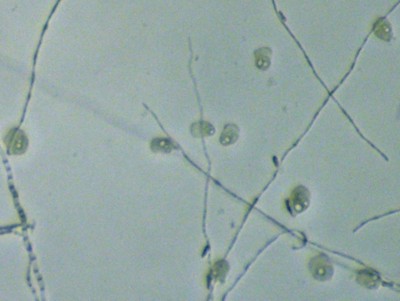The image appears to depict a microscopic view of a fluid containing several green cells, each with a small, see-through nucleus. The background is a whitish-gray, and multiple strands, resembling out-of-focus hairs, crisscross the scene in various directions, creating a mesh-like pattern. One strand on the left is slightly in focus, revealing a striated pattern of short horizontal stripes. The quality of the image isn't high, lending a somewhat hazy appearance to the objects. The cells, numbering around ten, are scattered sparsely and do not seem to be interacting with each other, floating independently within the solution.